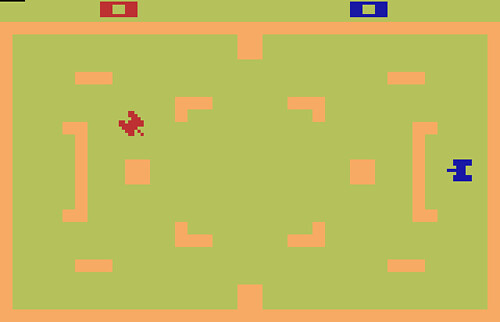This image is a screenshot from a vintage Atari video game that evokes the classic maze style of early arcade games like Pac-Man. The background features a light green color, and a peach-colored rectangular area appears in the center, resembling a maze filled with barriers. Within this maze, there are two primary competitors: a red one positioned on the left and a blue one situated on the right. The red player is located in the top left corner outside the maze, while the blue player is positioned similarly in the top right corner.

Inside the maze, the structure is comprised of intersecting lines that form pathways and obstacles, requiring the characters to navigate carefully to avoid collisions. The characters themselves are shaped like the letter "M," each with an antenna-like protrusion in the middle, giving them an appearance similar to classic video game controllers. The red character is oriented diagonally, pointing downward to the right, while the blue character is centrally located on the right side of the maze, pointing to the left. The intricate design and nostalgic elements make this screenshot a vivid representation of early video gaming aesthetics.